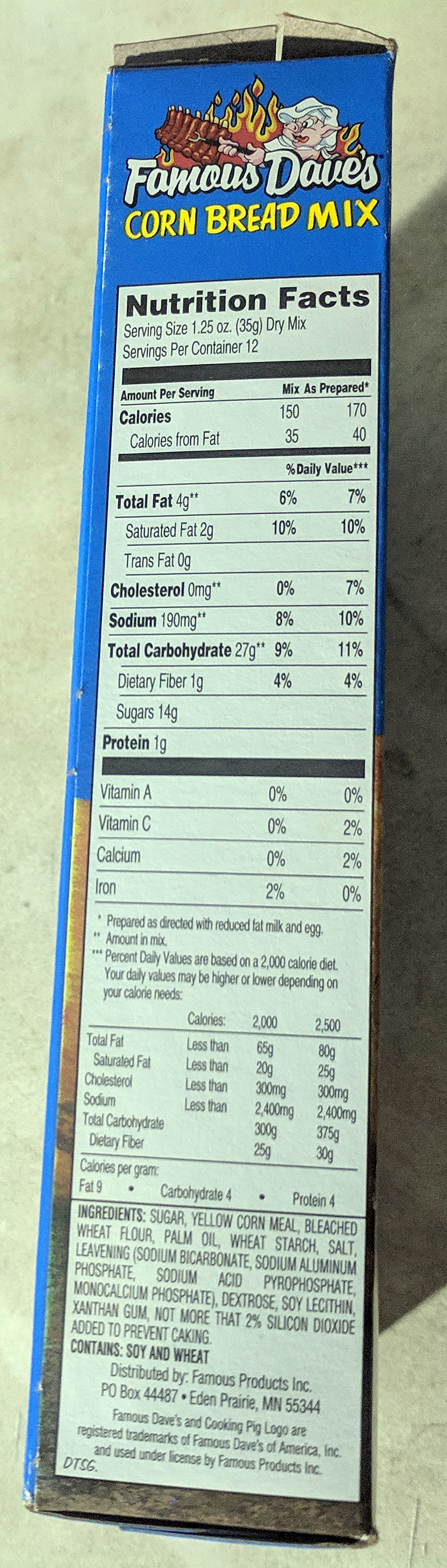This is a vibrant color photograph showcasing the side of a box of Famous Dave's Cornbread Mix. At the top of the box, the product name "Famous Dave's Cornbread Mix" is prominently displayed. Below the product name, a whimsical cartoon character of a pig dressed in a chef's hat and uniform is depicted, diligently cooking a rack of ribs over an open fire, adding a playful touch to the packaging.

Beneath the cartoon, the detailed nutrition label is clearly visible. The label provides the following information: 
- Serving Size: 1.25 ounces (35 grams) dry mix
- Servings Per Container: 12
- Calories: 150
- Calories from Fat: 35
- Total Fat: 4 grams
- Saturated Fat: 2 grams
- Trans Fat: 0 grams
- Cholesterol: 0 milligrams
- Sodium: 190 milligrams
- Total Carbohydrate: 27 grams
- Dietary Fiber: 1 gram
- Sugars: 14 grams
- Protein: 1 gram
- Vitamin A: 0%
- Vitamin C: 0%
- Calcium: 0%
- Iron: 2%

The ingredients list includes sugar, yellow cornmeal, bleached wheat flour, palm oil, wheat starch, salt, leavening agents (sodium bicarbonate, sodium aluminum phosphate, sodium acid pyrophosphate, monocalcium phosphate), dextrose, soy lecithin, xanthan gum, and up to 2% silicon dioxide to prevent caking. It notes that the mix contains soy and wheat.

The box is distributed by Famous Products, Inc., located at P.O. Box 44487 in Eden Prairie, Minnesota, 55344. It also mentions that "Famous Dave's" and the "Cooking Pig" logo are registered trademarks of Famous Dave's of America, Incorporated, and used under license by Famous Products, Inc.

This image is characterized by its significantly taller than wide aspect ratio, providing a full view of the product's side panel in a clear and detailed manner.